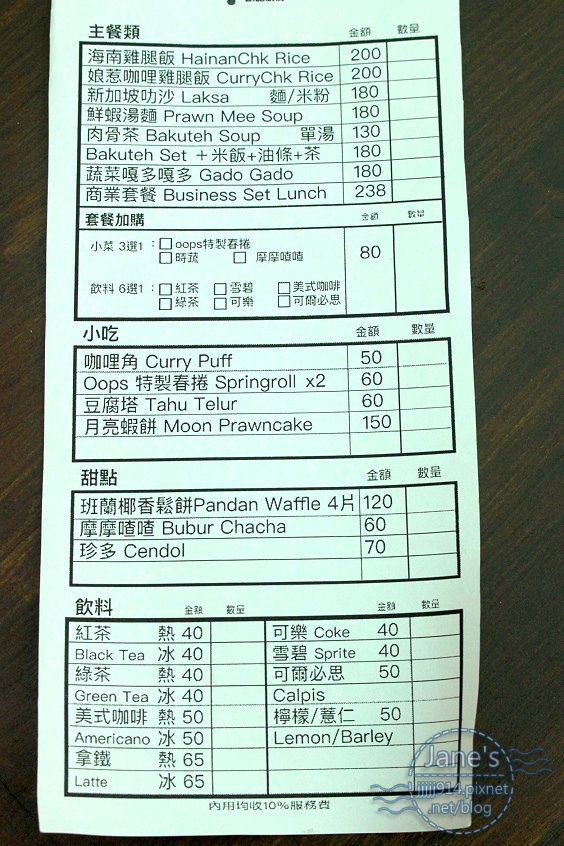The image captures a detailed photograph of a green restaurant menu, predominantly written in Chinese characters with corresponding translations and prices listed in Chinese yuan on the right. Set against a contrasting black background, the menu is divided into four sections. The top and largest section lists multiple entrees, including Hainan chicken rice, curry chicken rice, laksa, prawn mee soup, bakuda soup, bakuda set, gado gado, and a business set lunch, each accompanied by checkboxes for selection. Below, three smaller black boxes display additional food items and drinks with their respective prices: curry puff, spring rolls, tao chiller, moon prawn cake, pandan waffles, bubur cha cha, and sendol. Visible on the top right side of the photo is a logo reading "Jane's" followed by the URL jjjjj914.pixnet.net/blog.